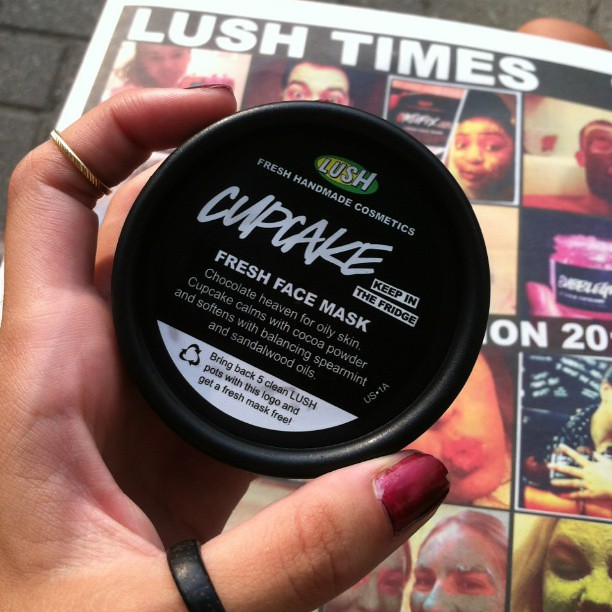An image depicts a woman's hand, adorned with a black ring on the thumb and a gold ring on the pointer finger, holding a black circular container. Her nails are painted in a deep red maroon color. The container features a green oval at the top with the white text "Lush Fresh Handmade Cosmetics." Below that, in a larger, more stylized font, it says "Cupcake." Two white horizontal bars read "Keep in" and "the Fridge." The label on the container further describes the product as "Chocolate Heaven for Oily Skin," noting that "Cupcake calms with cocoa powder and softens with balancing spearmint and sandalwood oils." At the bottom, another white bar states in black text, "Bring back five clean Lush pots with this logo and get a fresh face mask free." In the background, a colorful Lush Times newspaper advert shows various people wearing different colored face masks, including green, clear, and brown. Two girls are seen smiling with their face masks on, and a pink jar is also visible.